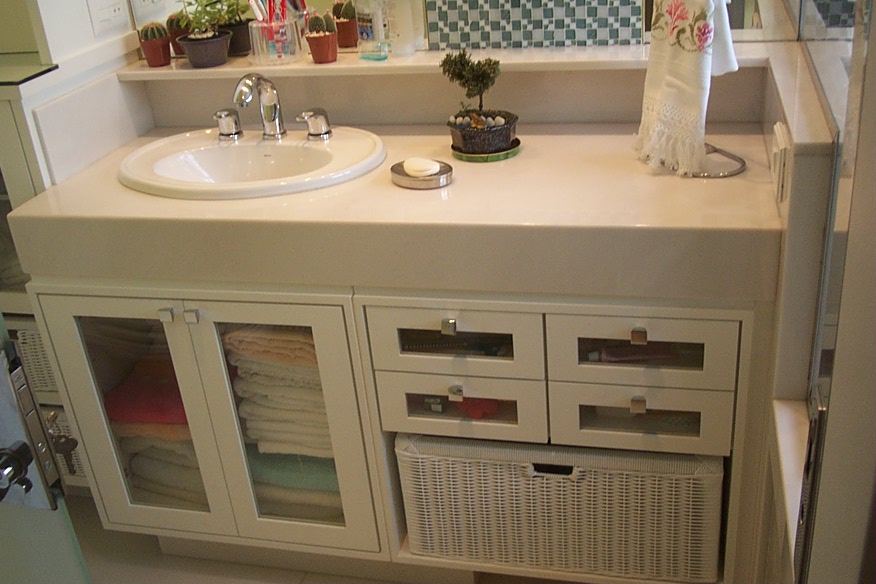This photograph showcases a meticulously organized bathroom sink area with several distinct elements. Central to the image is a ceramic bathroom sink equipped with a silver faucet and separate handles for controlling hot and cold water. Above the sink, a shelf houses a collection of small potted plants, including cacti, a bottle of mouthwash, and a jar containing toothbrushes, all of which are subtly reflected in the bottom of an out-of-frame mirror.

On the counter, to the left of the sink, there is a dish containing a bar of soap, positioned next to a small pot holding a bonsai tree. On the right, a standing rack adorned with a hand towel is placed in front of another shelf.

Below the sink, an unfilled area gives way to glass-fronted cabinets and drawers—two cabinets and four drawers in total. Positioned beneath these drawers is a large laundry basket. The floor is covered with gray tiles, completing the minimalist yet functional design of the bathroom space.